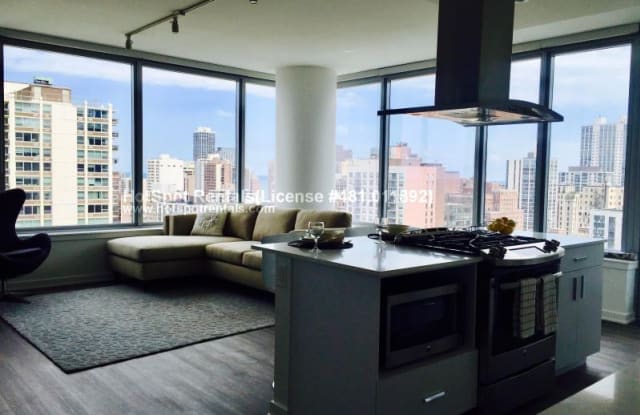In the high-rise living room, expansive floor-to-ceiling glass walls offer a breathtaking view of the cityscape, with numerous tall buildings dotting the horizon beneath a blue sky with scattered white clouds. The centerpiece of the room features a modern kitchen island, complete with a sleek stove and oven, flanked by cupboards on either side. Suspended above the stove is an elegant stainless steel vent. 

An L-shaped brown couch anchors the seating area, positioned on a large gray rug. A contrasting black chair enhances the cozy setup, inviting relaxation. A sturdy round pillar stands in one corner, providing structural support. Overhead, a sophisticated track lighting system with adjustable, round fixtures adds a contemporary touch, allowing for customizable illumination.

The floor is a sleek, wood-look laminate or possibly porcelain tile, adding to the overall stylish yet practical ambiance of this urban retreat.